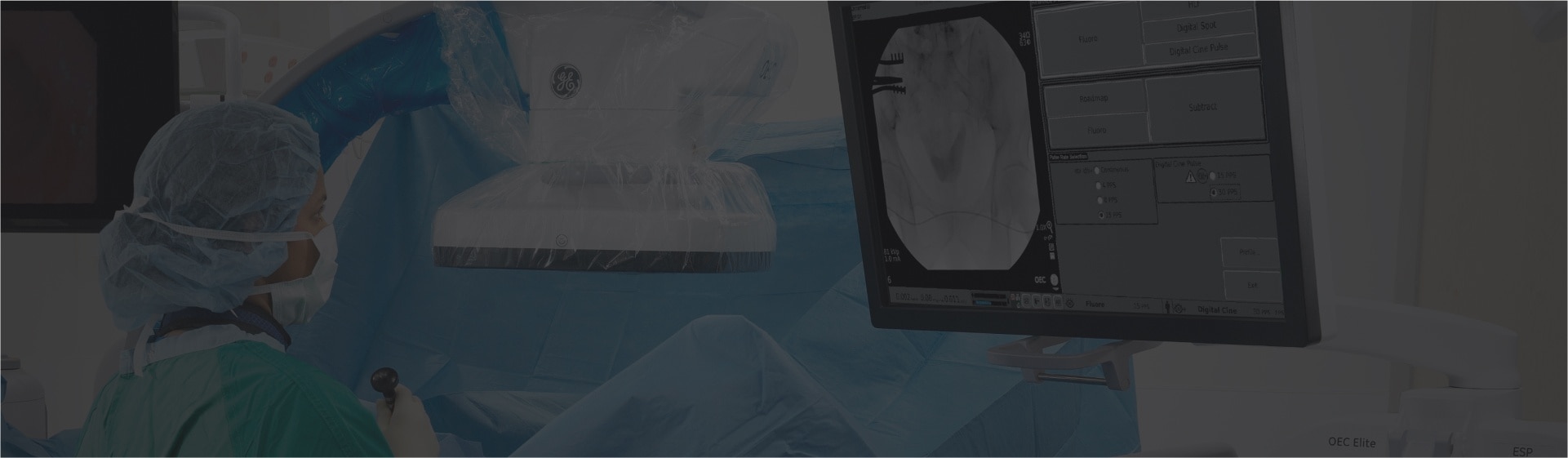In a low-quality photograph of a hospital surgery room, a female medical professional, identifiable by a surgical hairnet, green scrubs, white gloves, and a surgical face mask, is seen conducting a medical procedure. She appears to be using a large, white medical camera, which is covered with a clear plastic shield, to perform imaging on a patient. The camera is lowered down over a patient, who is partially visible and draped in a blue surgical cloth with knees propped up. The woman is holding a black joystick-like controller, maneuvering the camera, and examining the resulting images on a nearby monitor. The monitor displays the ongoing procedure, while the background of the room is cluttered with hospital linens and equipment shrouded in protective coverings, maintaining the sterile environment.